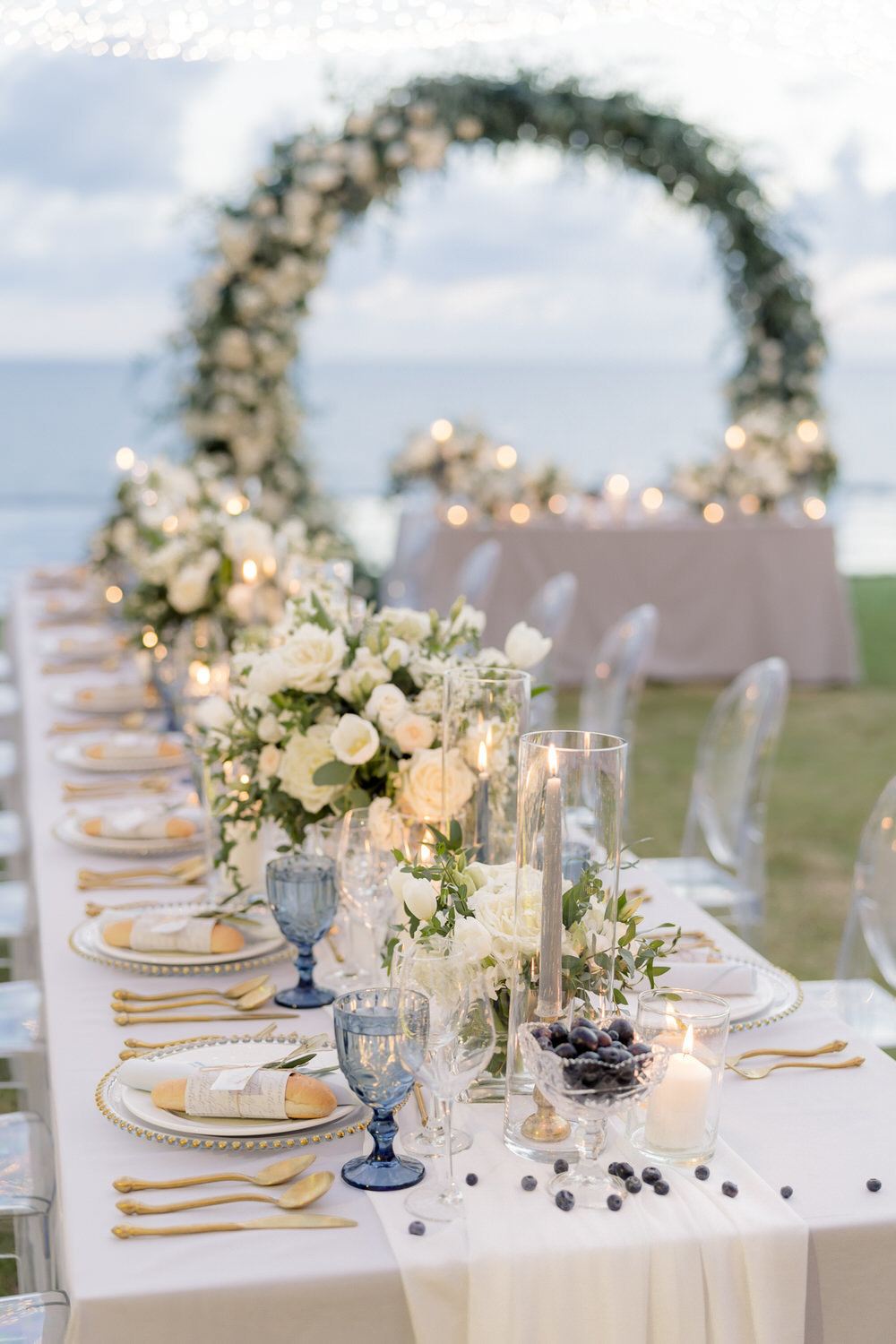This image captures an exquisite wedding reception set outdoors on a picturesque beach. A long banquet table, elegantly dressed in a white tablecloth that drapes like a regal gown, is prominently featured. The table is meticulously set with golden silverware including spoons, forks, and knives, contributing to the overall fancy and regal ambiance. Blue glass goblets and candles add a touch of sophistication, while an unusual yet charming sprinkle of blueberries decorates the table.

Centered in the image, the banquet table extends to the left, adorned with an abundance of white flowers and further embellished with beige and whitish floral arrangements. The head table is slightly blurred in the background, sitting under a lush floral archway filled with green leaves and soft pastel flowers, signaling where the wedding party might be seated.

Flanking the table on the right is a display featuring a beige tablecloth, lit candles, and additional floral decorations, while white and gold-trimmed chairs are arranged on the left. Each plate, also trimmed in gold, holds a ready-to-eat breadstick, emphasizing the well-thought-out and luxurious details of the setting, indicative of a celebration where no expense was spared.